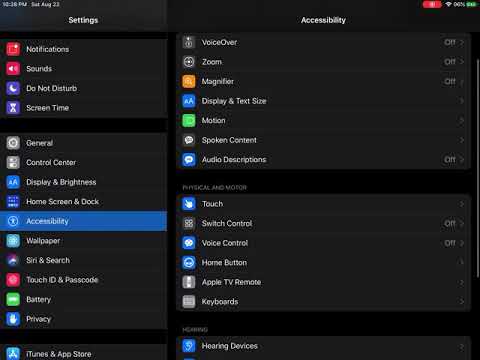This image is a detailed screenshot of the "Settings" page on a tablet device, likely an iPad, characterized by a black background. The screen is divided into two primary columns. The left column is the main navigation pane for the settings, organized into several sections. The first section includes options for "Notifications," "Sound," "Do Not Disturb," and "Screen Time." Below that, the next section features "General," "Control Center," "Display & Brightness," "Home Screen & Dock," and "Accessibility," with "Accessibility" highlighted in blue, indicating that it is currently selected. Further down, this section lists "Wallpaper," "Search," "Touch ID & Passcode," "Battery," and "Privacy," with another section cut off at the bottom starting with "iTunes & App Store."

The right column showcases the "Accessibility" settings in detail. This larger pane lists numerous options with colored icons next to each, such as "VoiceOver," "Zoom," "Magnifier," "Display & Text Size," "Motion," "Spoken Content," "Audio Descriptions," under a section for visual accessibility options. Another section includes options like "Touch," "Switch Control," "Voice Control," "Home Button," "Apple TV Remote," "Keyboards," and finally, at the very bottom, "Hearing Devices." All these options indicate various on or off states, visually represented by switches next to each.